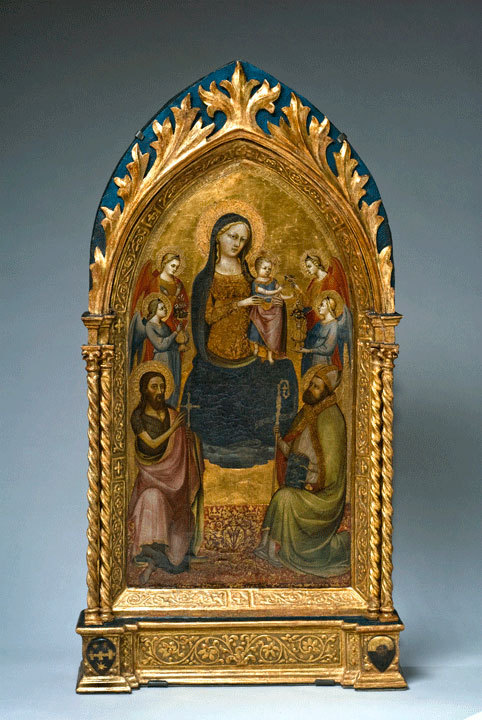The photograph is of an intricately detailed, arched Christian religious artifact, likely meant for display on an altar. The panel is opulently gilded with gold foil texture and decorations, and features a medieval Italian painting circa 1410. The central focus is the Virgin Mary clothed in a blue dress, holding the infant Jesus. Surrounding them are four angels, two on each side, and two saints kneeling at the base; the saint on the right dons a green robe and hat, while the saint on the left wears a red robe and holds a cross. The golden arch, pointed at the top, is adorned with elaborate flourishes and set against a gray wall, emphasizing its rich, shimmering quality. The scene within the arch is framed by vibrant hues and detailed medieval artistry, showcasing the holiness and reverence of the figures depicted.